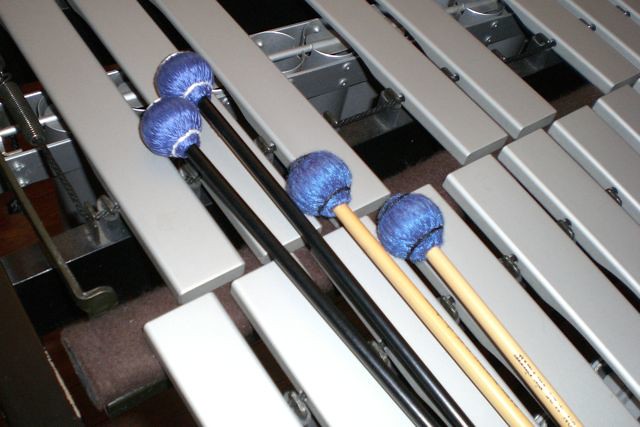The image showcases a detailed, zoomed-in portion of a xylophone with light gray, rectangular metal bars arranged in two rows. The bottom row contains around 10 to 15 keys stretching from the left corner to the right, while the top row has fewer keys, with noticeable gaps. There are four mallets placed on the xylophone; two have natural wood-colored sticks with blue spherical heads, and two have black sticks with the same blue heads. The frame of the xylophone is partly visible, displaying a black section, and there are cylindrical objects under the keys along with a purple fuzzy border. The background features slight portions of a brown floor and a hint of black at the top.